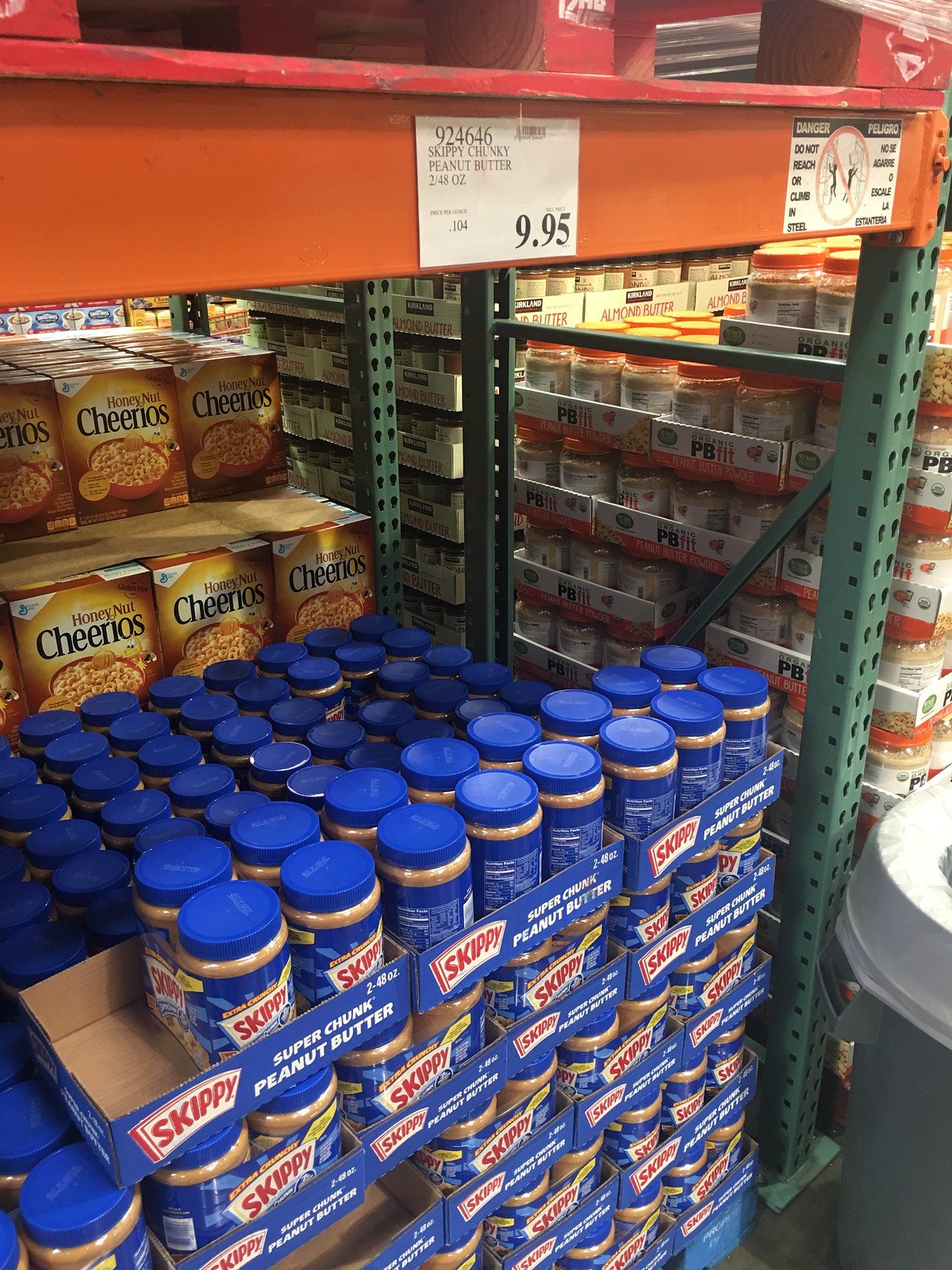The photograph captures the interior of a well-known warehouse club store, likely a Sam's Club or Costco, where items are sold in bulk quantity. Dominating the image are multiple pallets loaded with giant two-packs of Skippy Super Chunk peanut butter, distinguished by their blue plastic lids. A prominent price tag above the stacked pallets reads, "Skippy Chunky Peanut Butter, 2/48-ounce, $9.95." Behind these are towering pallets of Honey Nut Cheerios, housed in their characteristic golden-yellow boxes featuring a bowl of cereal on the front. To the right of the peanut butter, another pallet is stocked high with jars of PB Fit peanut butter powder, noticeable by their orange lids. The items are placed on heavy-duty metal shelving, emphasizing the bulk-shopping nature of the store, where customers and small business owners can purchase large quantities of goods.